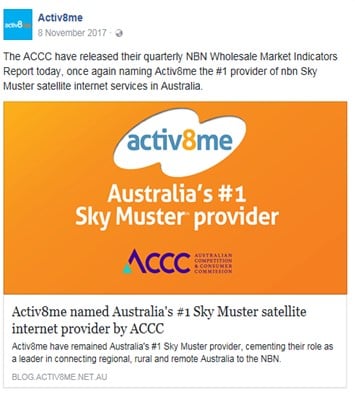This image appears to be a screenshot of an advertisement or announcement. 

At the top, there is a username, formatted as "ACTIV8ME," followed by the date, "8 November 2017." The main content is placed against a white background with black text, featuring a paragraph announcing that the AACCC has released their quarterly NBN Wholesale Market Indicators report. This report names ActivateMe as the number one provider of NBN SkyMuster satellite internet services in Australia.

Below the paragraph, there is an orange rectangle containing the text "ActivateMe" with the tagline, "Australia's number one SkyMuster provider," written underneath. 

Additionally, there is a reference to the AACCC, although some of the lettering is difficult to read. Further down, there is another block of text on the same white background, reiterating that ActivateMe has been named Australia's number one SkyMuster satellite internet provider by the AACCC. It also highlights ActivateMe's continued leadership in connecting regional, rural, and remote areas in Australia to the NBN.

At the very bottom left corner, in greyed-out lettering, the text "blog.activateme.net.au" is visible, likely indicating the source or further information.